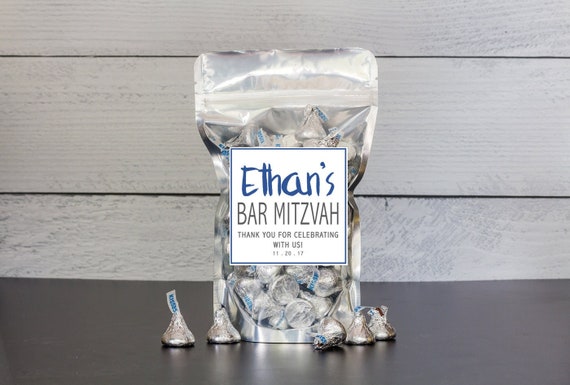The image showcases a party favor from Ethan's Bar Mitzvah, held on November 29, 2017. It features a clear, see-through bag filled predominantly with silver-wrapped Hershey's Kisses, along with five individual kisses placed in front of the bag. The bag has a custom label stating, "Ethan's Bar Mitzvah, thank you for celebrating with us", and includes the date. The favor is presented on a dark brown table, set against a whitewashed or light gray paneled wall. The bag appears to have a reusable seal at the top. The product is centrally framed and, while slightly blurry, provides a clear view of the festive packaging and the accompanying chocolates, creating a memorable keepsake from the celebration.